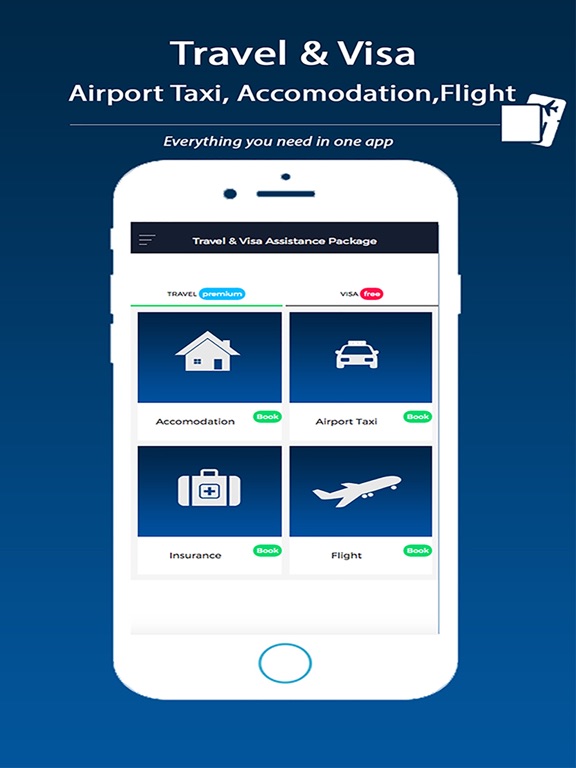This image, sourced from a travel and visa assistance website, details a comprehensive app designed to streamline travel planning. The upper section of the image introduces the app's all-inclusive features, highlighting its capabilities for handling airport transfers, taxi services, accommodations, and flights.

Prominent on the left side is a labeled image of a house, signifying the accommodation booking feature, with a noticeable green "Book" button adjacent to it. To the right, the app's airport taxi service is represented by an image of a taxi cab, also accompanied by a green "Book" button. 

Below the taxi service, on the left, is an insurance booking option marked by an image of a first aid kit and another green "Book" button. On the far right, an illustration of a large airplane signifies the flight booking service, situated above a corresponding green "Book" button.

The app offers various packages tailored to different travel needs, such as a travel and visa assistance package, a travel premium package, and a visa-free package, ensuring a wide range of services are covered for the user.